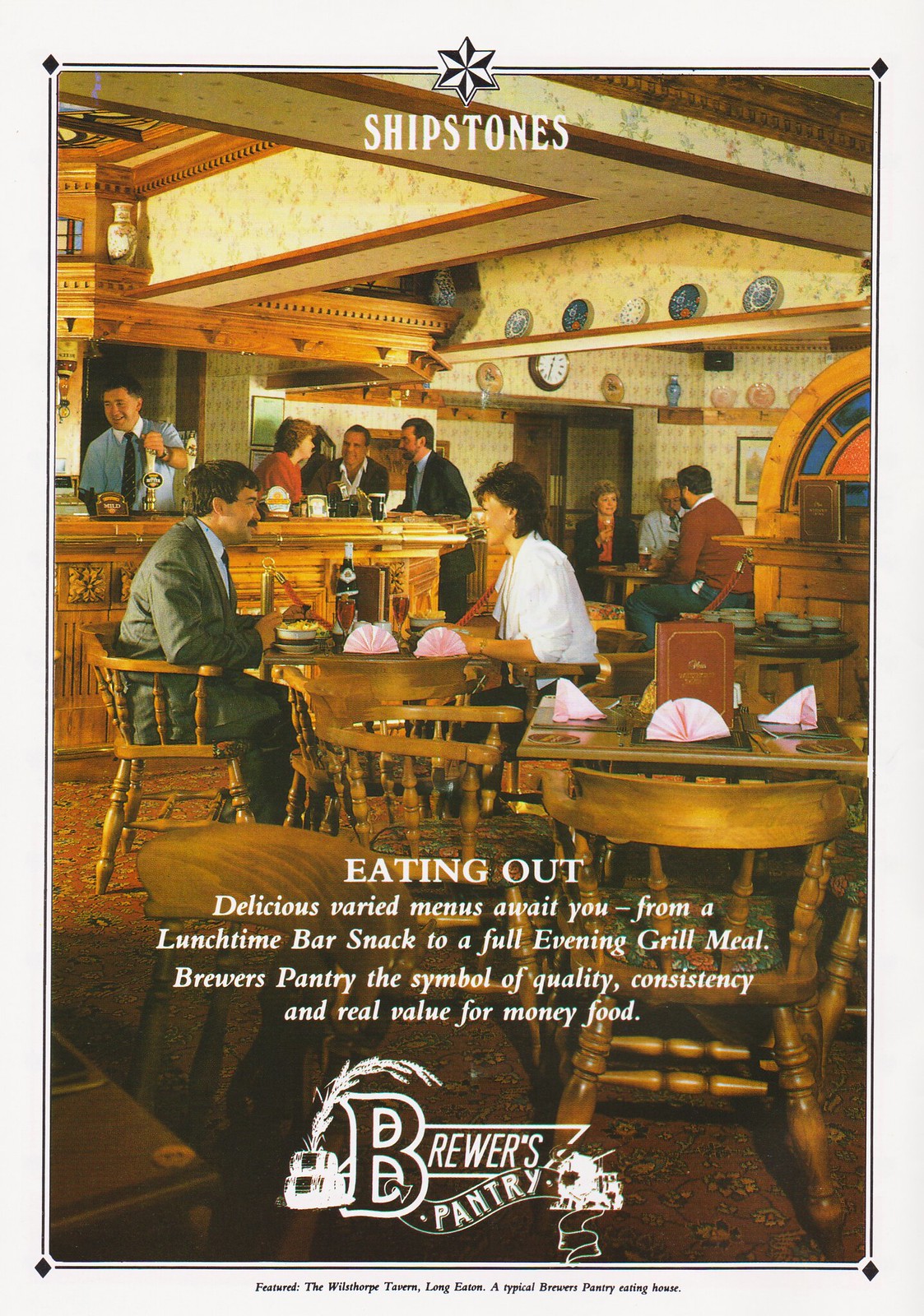The promotional poster for Brewer's Pantry features a photograph of a warm, inviting bar or tavern dining area, framed by a gray border with black diamond shapes in the corners. The center image showcases multiple square-shaped tables, each accompanied by four round wooden armchairs that have green seat cushions. Every table is set with a red menu, four placemats, and pink napkins folded into fan shapes. The decor predominantly features wood and traditional wallpaper, suggesting an older, classic ambiance. 

In the restaurant scene depicted, there are various groups of patrons: a man in a brown suit and a woman in a white shirt are conversing at a table towards the center, while in the foreground, three people sit together, engaged in conversation. Additionally, two groups of three are visible—one at the bar and another at a table in the back. A bartender is seen interacting with customers behind the bar. The floor is carpeted in brown with a design that complements the wooden furnishings.

Text overlaid on the image advertises "Ship Stones" at the top, accompanied by a star, and at the bottom it reads, "Eating out. Delicious varied menus await you, from a lunchtime bar snack to a full evening grill meal. Brewer's Pantry, the symbol of quality, consistency, and real value for money food." The Brewer's Pantry logo appears at the bottom of the poster, reinforcing the establishment's commitment to excellent dining experiences. Additionally, the poster features barrels with barley sprouting from them, enhancing the rustic and authentic vibe.